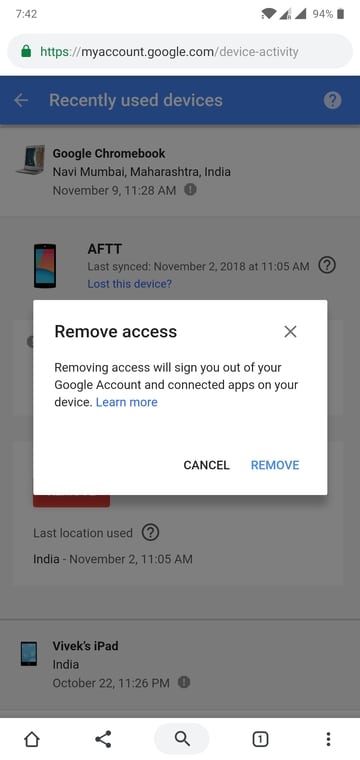In this screenshot, we observe various details across the user interface of a mobile device. At the top of the screenshot, the current time reads 7:42 AM. Adjacent to the time on the upper right, there is a Wi-Fi signal icon displaying four bars, indicating a strong connection. Next to it are two network signal bars, where the first bar is not fully filled, and the second bar is completely filled. Furthermore, the battery level indicator is visible, showing the device battery at 94%.

The central part of the screenshot contains text with specific details. It reads "Google Chromebook, Navi, Mumbai, Maharashtra, India." Below this, further details mention "November 9th, 11:28 AM, AFTT." Additionally, there's information about the last synchronization, "last synced, November 2nd, 2018, at 11:05 AM." 

There is a message indicating the removal of access, along with the implications: "Removing access was signing out of a Google account and connected apps on the device." Options presented include "Learn more," "Cancel," and "Remove." 

Towards the bottom, another device is listed: "Vivek's iPad, India, October 22nd, 11:26 PM." This comprehensive collection of details provides a clear and thorough overview of the pertinent information contained in the screenshot.